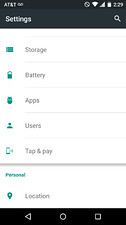This image is a small vertical rectangular photo, capturing a screenshot of a phone's settings page. The screenshot features a thick black border at the top and a thinner black border at the bottom. Within the top black border, on the right side, there are several icons. The far-right icon shows the time, immediately followed by the battery icon, the signal strength icon, and finally, a WiFi icon from right to left. Additionally, at the very top left within this black border, the network provider "AT&T" is displayed in white text, accompanied by a voicemail icon that resembles a small tape next to it.

The predominant body of the screenshot is a white background displaying various settings options. The visible settings categories include "Storage," "Battery," "Apps," "Users," and "Tap & Pay." Towards the left side of the screen, the word "Personal" is highlighted in blue, with the "Location" setting listed below this category. 

At the bottom of the screenshot, there is a navigation bar featuring three icons: a left-pointing triangle on the left, a circle in the center, and a square on the right side.